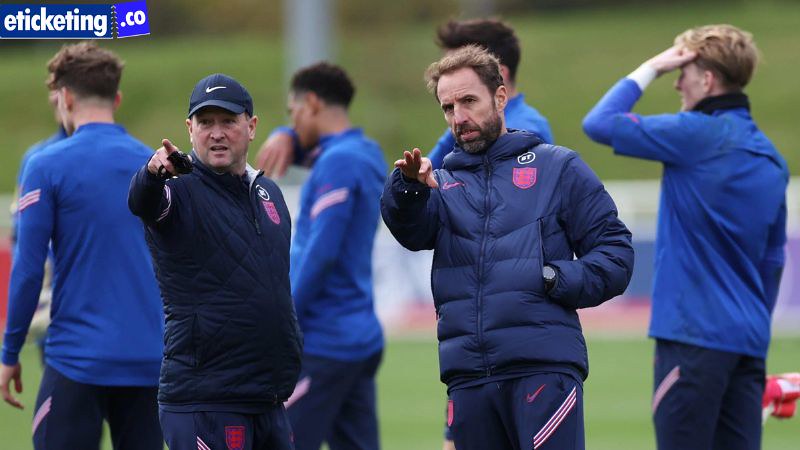The photograph captures a moment on a soccer field, where a group of men appear to be engaged in a team gathering or strategy session. The flat, green field is bordered with railings adorned with banners, setting a slightly overcast ambiance. Prominently in the top left corner, a blue banner emblazoned with "e-ticketing.co" adds a splash of color against the muted sky.

Five younger players, dressed in light blue shirts and navy blue pants with red and white markings, stand lined up in the background, seemingly worn out and fatigued; one of them has a hand on his forehead, possibly in frustration. In the forefront, two men—likely coaches—are seen in blue pleated jackets and matching blue pants with red stripes. The coach on the left wears a zippered jacket and a blue baseball cap featuring a white Nike logo. Both coaches seem to be pointing and directing attention to something off-screen to the top left, perhaps discussing tactics or observing an ongoing event. The scene, characterized by the coaches' apparent strategizing and the players' exhaustion, hints at the demanding nature of the sport and the relentless pursuit of improvement.